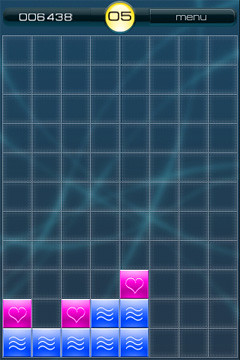The image is a vertically aligned screenshot of a Tetris-style video game displayed in portrait mode, possibly taken from a smartphone app. The background features a smoky blue color with a grid pattern composed of light blue lines forming squares. At the bottom left, there are eight cubes in total. Five of these cubes are blue with three vertically stacked wavy white stripes and three heart-shaped pink cubes positioned above the first, third, and fifth blue cubes. The fourth and fifth cubes have additional blue ones on top, with the fifth cube also supporting a pink heart cube. At the top of the screen, the game interface displays the menu button on the right and a number sequence "006438" on the left. Centrally aligned at the top, there's a gold circle with a black border containing the number "05."